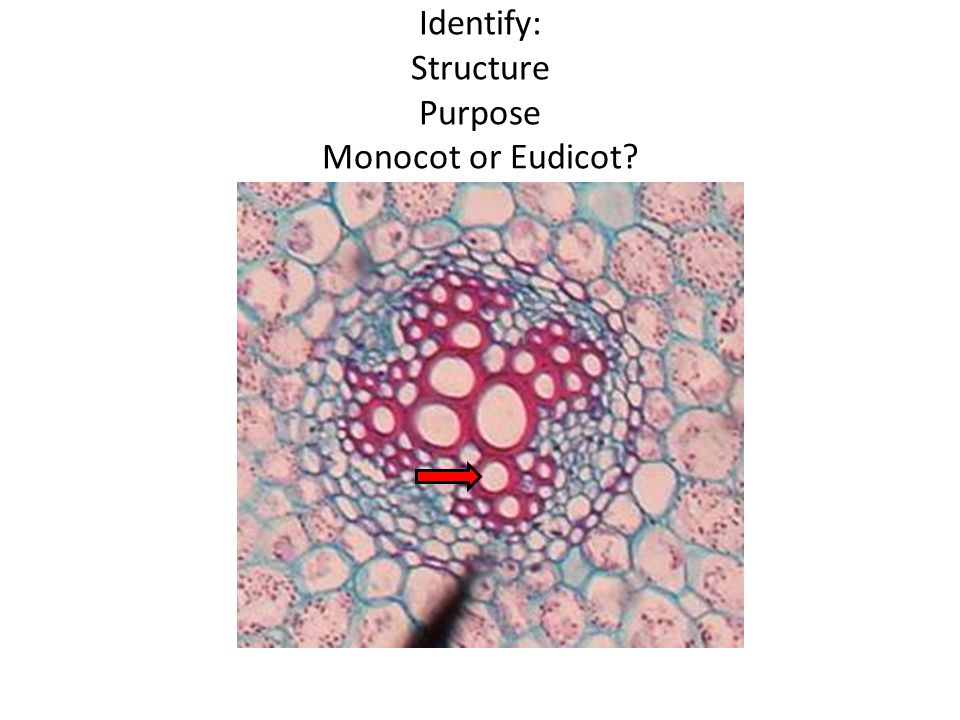The image appears to be a highly magnified view of a group of cells, likely captured for educational purposes, such as a medical or biology class. The top of the slide bears text instructing viewers to "identify the structure, purpose, monocot or eudicot," suggesting a focus on plant cell classification and structure. The cells are predominantly rounded and centrally located, exhibiting a variety of colors including peach, light blue, purple, and varying shades of pink and magenta. The middle of the image features a cluster of cells with white centers and magenta linings. Surrounding this central cluster are larger reddish cells, encased by purplish-banded cells and further enclosed by larger cells with a bluish tint. These visual cues point to an intricate arrangement possibly highlighting different cellular components or conditions, serving as an essential reference for university students or individuals studying cell biology.